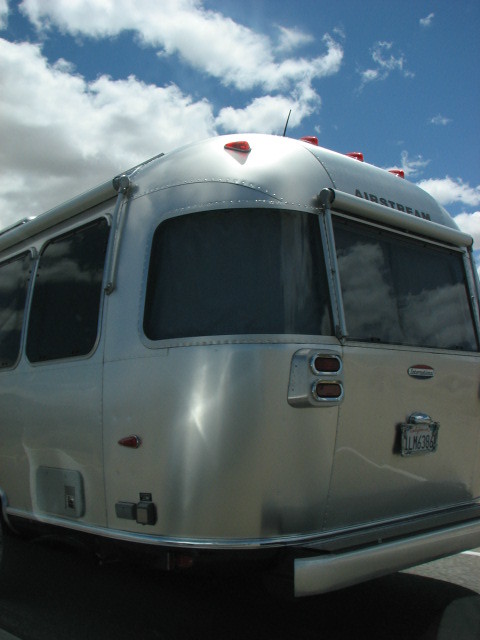This outdoor photograph captures a retro-styled, metallic silver Airstream vehicle, prominently positioned at the center. The sky above is a rich blue, scattered with clouds, indicating it was taken during the day. The vehicle sits on an asphalt road, enhancing its chrome-like sheen. 

Airstream is clearly inscribed in dark grey letters above the rear window. Below this window, the license plate reads LM6386, and directly beneath that is a silver bumper, matching the vehicle's metallic exterior. The retro sci-fi aesthetic is accentuated by visible bolts along the metal panels. Red lights adorn the top and sides of the Airstream, including distinct reverse and brake lights on the back. Black-framed windows run along the vehicle's sides, though they offer limited additional details.

Moreover, the vehicle features a retracted awning on its side and apparent power plugs, contributing to its functional aspects. The photo conveys a nostalgic, futuristic vibe with its polished, streamlined look.